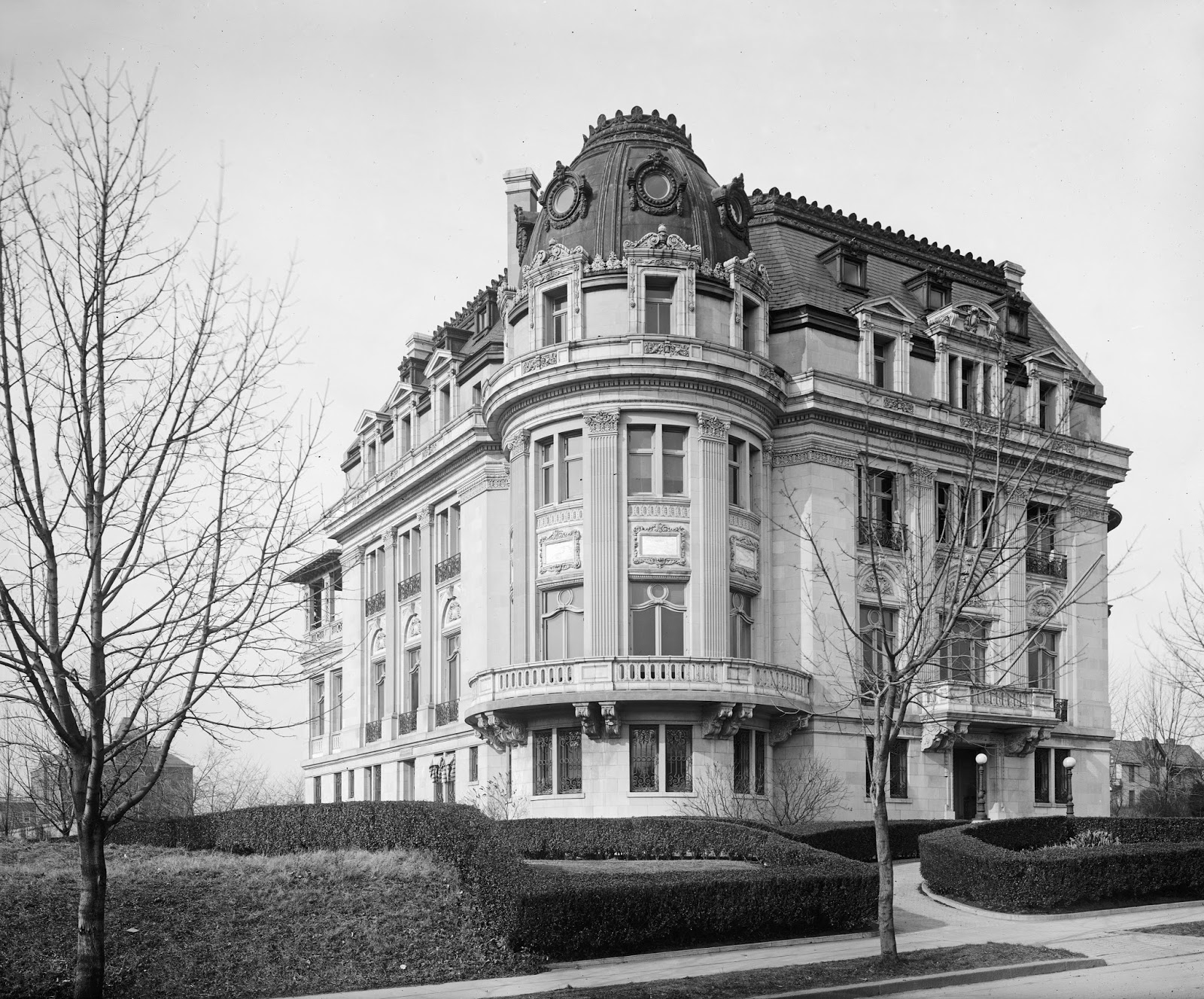The black-and-white photograph captures a corner side view of a grand, five-story Victorian mansion complete with an attic. Prominent features include a turret-like rounded corner crowned with a dome-like roof, and numerous well-designed windows, including several attic windows. The mansion stands out with its white stone facade and darker roof. In front, a meticulously landscaped garden with well-manicured flowers and hedges graces the yard, along with a circular driveway leading to a sidewalk. The scene is framed by two bare trees, indicative of winter. Additional details reveal a front door flanked by lampposts and a top balcony with stone railings that wraps around the turret. In the distant background, two smaller buildings are faintly visible.